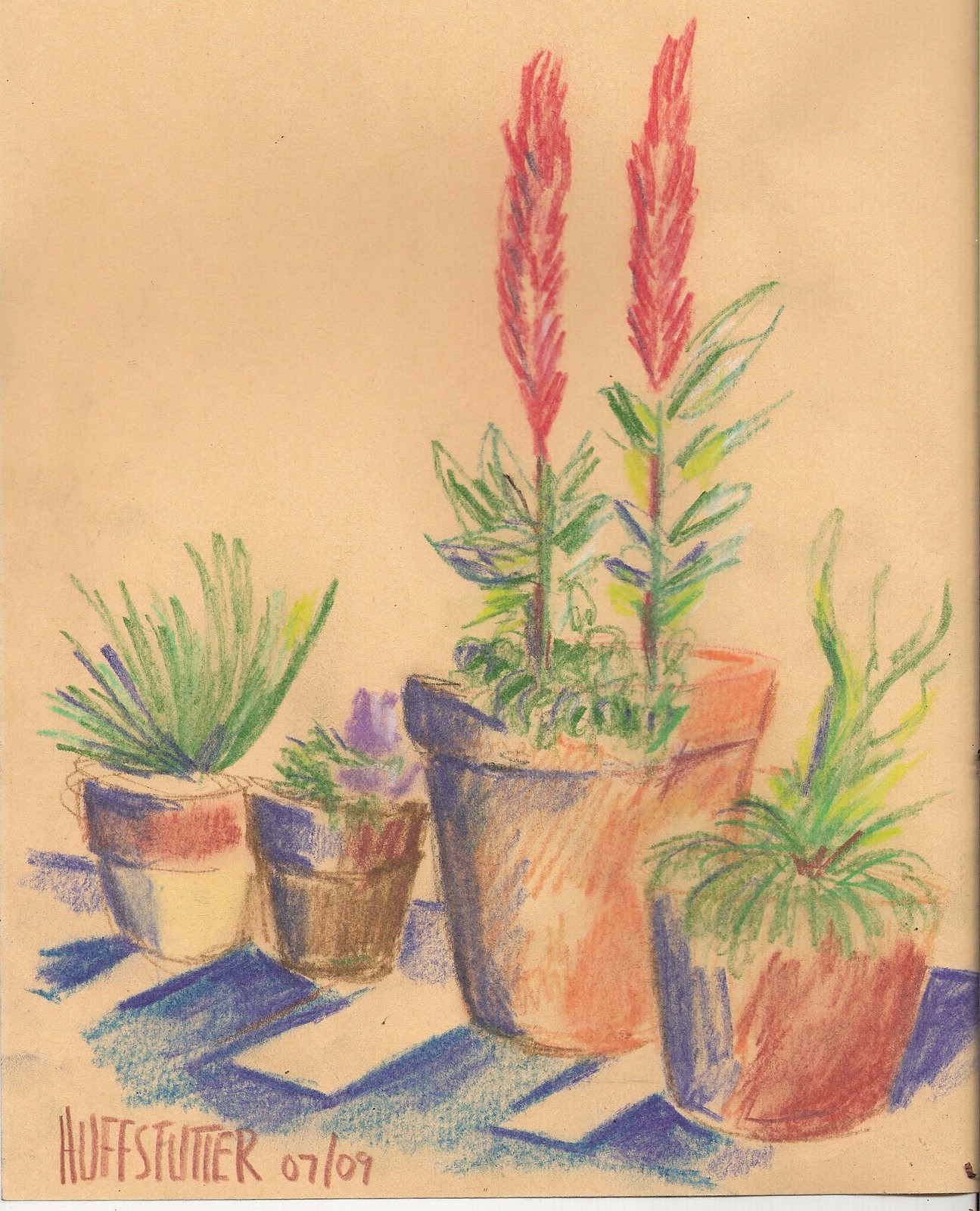This artwork features a hand-drawn illustration of four potted plants rendered on a beige-tan paper, lending a vintage and textured feel to the piece. The illustration seems to be created with colored pencils or crayons, given the rough, textured appearance of the strokes. At the bottom left corner, the words "Huffstudio 0709" or "Huffstoyter 0709" are inscribed.

The largest plant, located third from the left, stands out with its two vertical pink flowers and green leaves, providing a vibrant focal point. The other three plants, which are smaller in size, include a variety of greenery and flowers: from line-drawn leaves to green succulents. One of these smaller plants appears to have a wispy, red feather-like flower, while another features a delicate purple bloom.

These terracotta and brown pots are arranged on a blue and white checkered surface, adding a rustic charm to the visually appealing composition. Scattered white spaces within the blue ground mimic the natural gaps commonly seen in sketches, enhancing the overall artistic and relaxed feel of the scene.